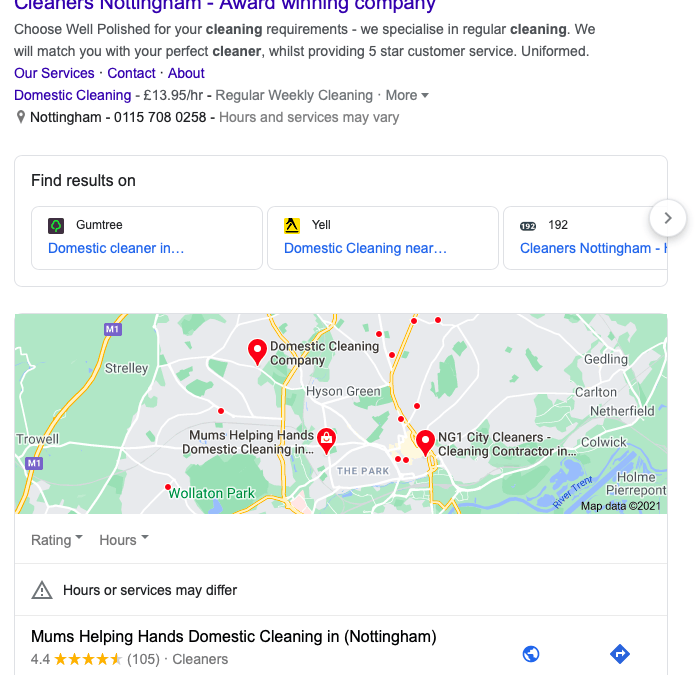This image depicts a search for domestic cleaning services in Nottingham. The search results prominently highlight an award-winning company titled "Cleaners Nottingham," shown in blue. Directly underneath, it states: "Choose Well Polished for your cleaning requirements. We specialize in regular cleaning. We will match you with your perfect cleaner whilst providing five-star customer service." The phrase "uniformed" is mentioned alongside information about their services, which include domestic cleaning at a rate of £13.95 per hour. Detailed contact information and a "more" button are provided, suggesting further details about regular weekly cleaning services. 

The image also indicates that search results can be found on platforms such as Gumtree, Yell, or 192. The map portion of the search results, taken from Google Maps, shows the location of the domestic cleaning company around Wollaton Park. It also marks the locations of "Mums Helping Hands Domestic Cleaning" and "NG1 City Cleaners," a cleaning contractor.

The listing for "Mums Helping Hands Domestic Cleaning in Nottingham" includes a 4.4-star rating based on 105 reviews, with additional information accessible by clicking on it. The note at the bottom advises that hours and services may vary.